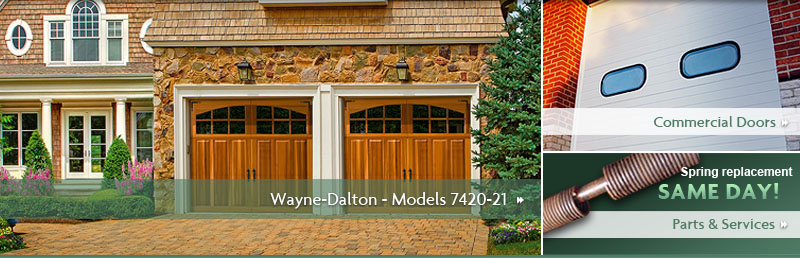This advertisement features three vibrant color images highlighting different types of garage doors and services. The prominent image on the left captures a close-up view of an elegant residential setup, showcasing two premium wooden garage doors from Wayne Dalton, model 7420-21. The house itself is exquisitely designed with stone surfaces, flanked by well-maintained landscaping that includes neatly trimmed bushes, two decorative small trees, and vibrant pink flowers flourishing around the front door. Above each garage door, modern light fixtures add a touch of sophistication to the overall aesthetic. 

To the right, a smaller image labeled "Commercial Doors" depicts a sturdy freight door, ideal for businesses or warehouses. The white door, equipped with two small blue-tinted windows, seamlessly fits into the red brick building, suggesting a combination of durability and functionality.

The bottom image, captioned "Spring Replacement - Same Day Parts and Services," presents a clear view of a garage door spring. The illustration is set against a green backdrop, highlighting a brown-colored garage door spring, emphasizing the availability of prompt repair services. This triptych effectively showcases a range of products while underscoring quality and attentiveness to detail.